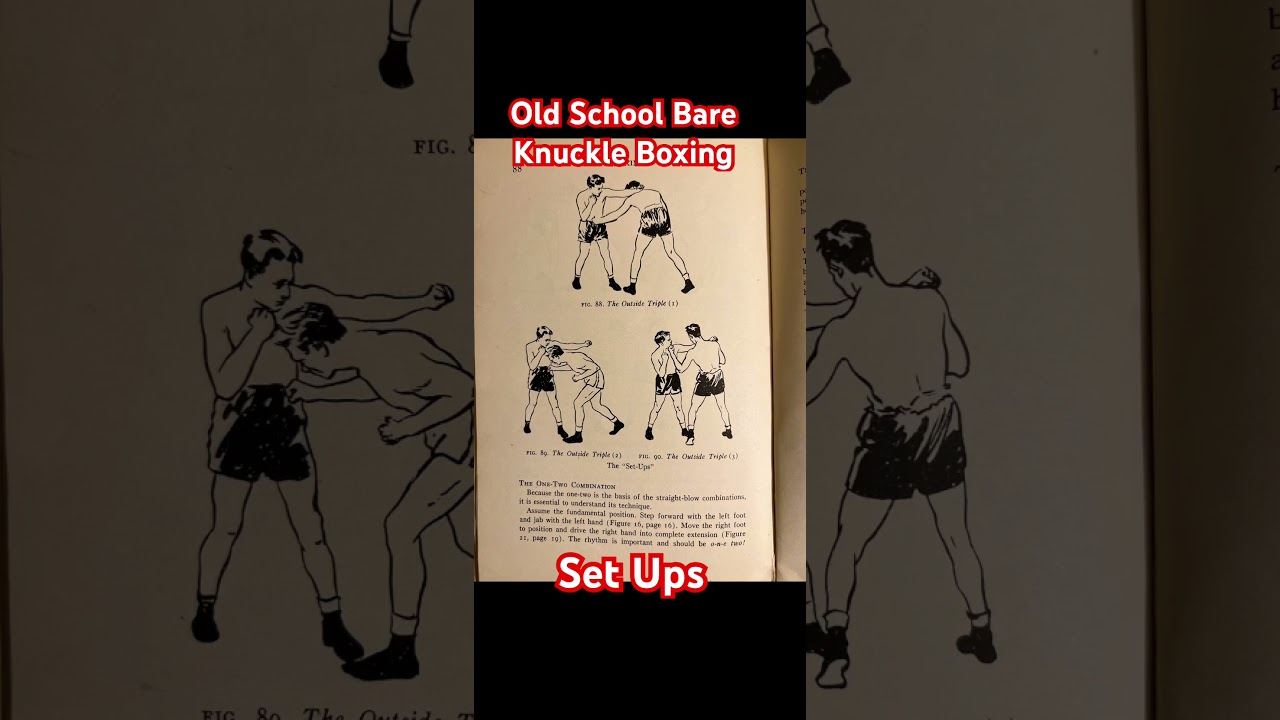The image depicts an instructional page from an old book or magazine on bare-knuckle boxing, emphasizing setups for the "outside triple" technique. The top of the page features the title "Old-School Bare-Knuckle Boxing" in white lettering on a red background, while the bottom reads "Setups" in similar style. The page number, 88, is marked at the top left. There are three pencil-drawn figures illustrating different stages of the "outside triple" combination. The top image, labeled "Figure 88: The Outside Triple," shows one man punching another in the stomach while the latter aims a punch towards his opponent's neck. The subsequent illustrations continue to describe the "outside triple" sequence, with detailed images of the one-two punch combination. This old instructional material provides a glimpse into traditional bare-knuckle boxing techniques, which are rarely practiced today without modern gloves and padding.